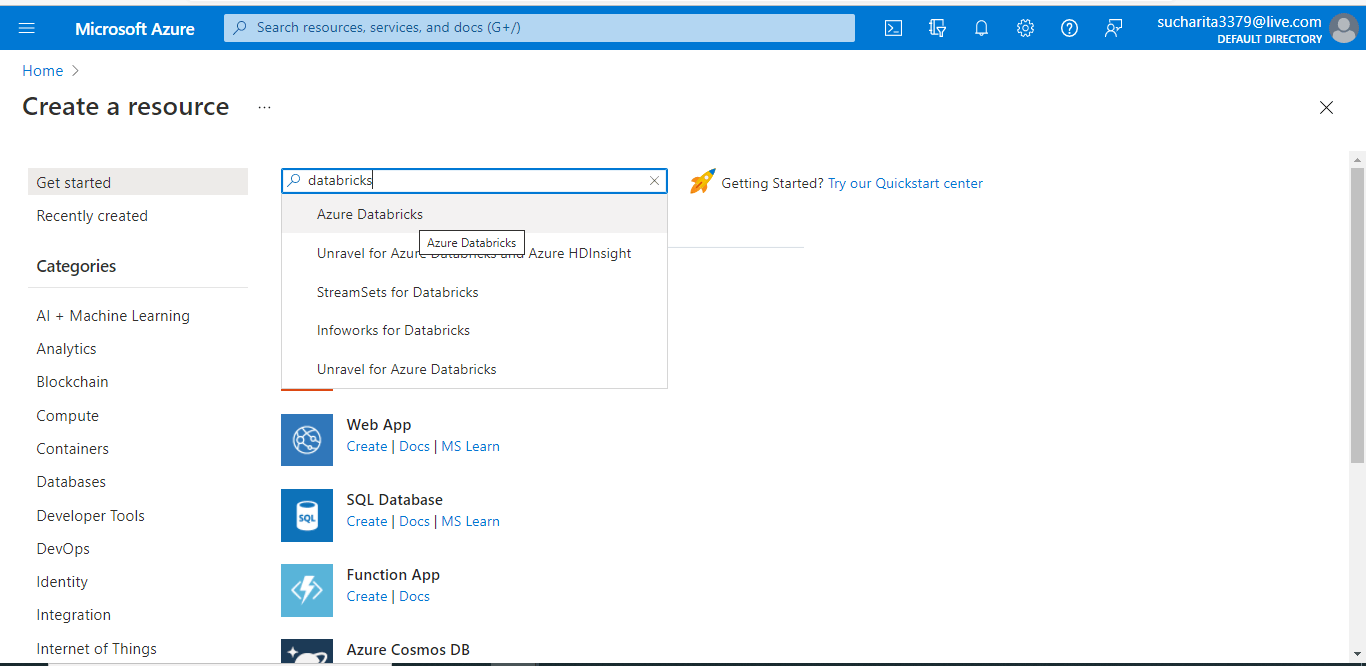This image is a detailed screenshot from the Microsoft Azure interface. The screenshot is horizontally oriented and features a distinctive blue navigation bar at the top. In the upper left corner of this bar, the text "Microsoft Azure" is prominently displayed next to an unutilized search bar.

Below the navigation bar, the screen transitions into a predominantly white space bordered subtly on the right side and bottom edge, hinting at the confines of the rectangle. In the upper left quadrant of this section, there's a heading that reads "Create a Resource," followed by an indication that the user has clicked on "Get started." A search box appears to the right, into which the term "Databricks" has been typed. This search yields a result labeled "Azure Databricks."

Further down the interface, there are several square icons arranged vertically. The first square is blue and labeled "Web App," featuring an image that resembles a ball. Directly below this, another blue square displays the text "SQL Database" alongside an icon that looks like a cup. The screenshot effectively showcases steps within Microsoft Azure's resource creation process, highlighting user interaction with search functionality and available service icons.